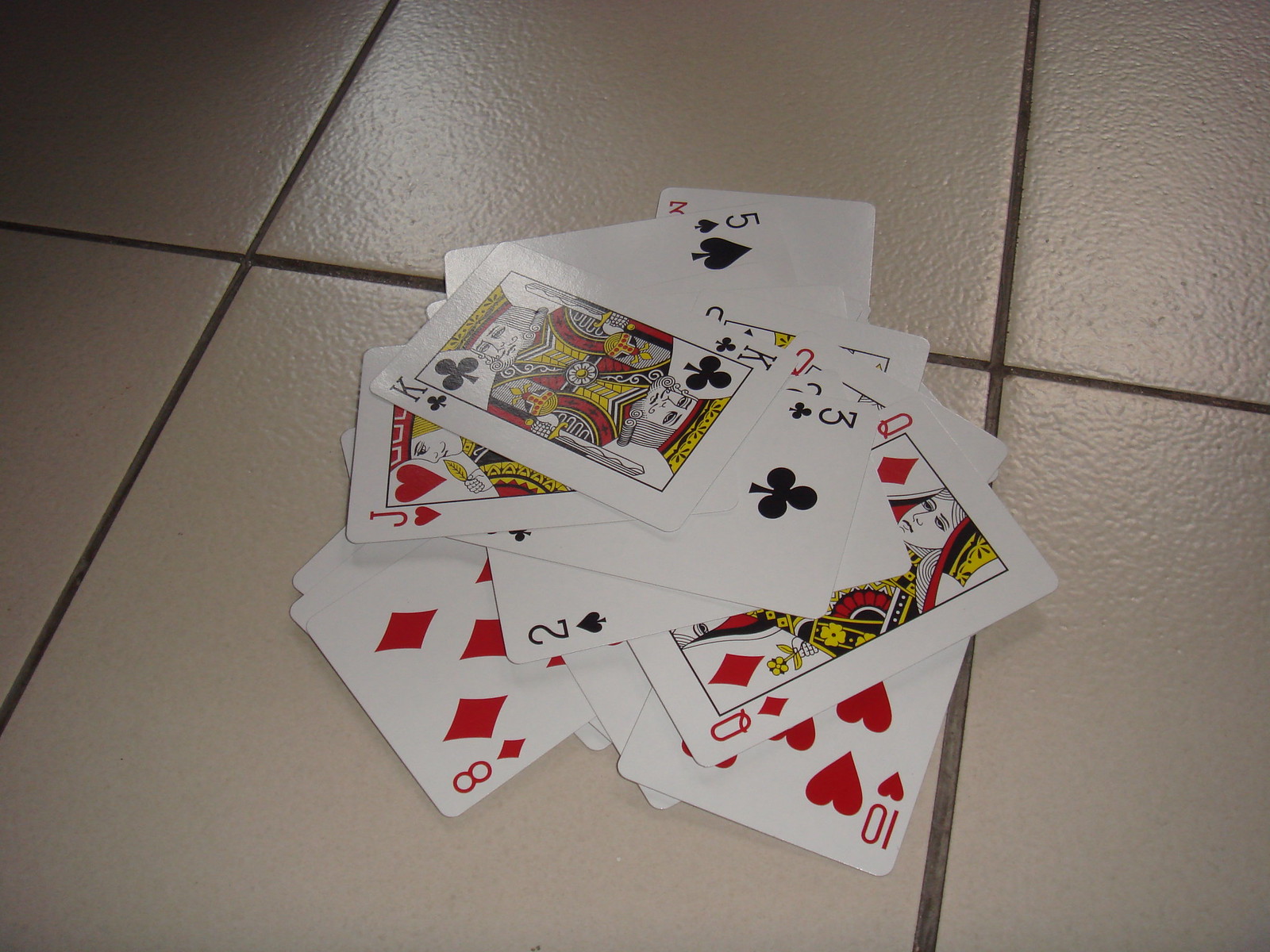A deck of playing cards lies scattered in an artful disarray on a tan tile floor, creating an impression of intentional rhythm rather than random chaos. The entire or nearly entire deck appears to be involved, with all visible cards face-up, revealing their suits and values. Among the spread, distinct cards such as the King of Clubs, Jack of Hearts, Three of Clubs, Two of Spades, Five of Spades, Eight of Diamonds, Queen of Diamonds, and the Ten of Hearts can be identified. Additionally, there is a Queen of Hearts, recognizable by its red suit. One card remains ambiguous, showing only a '3', suggesting it is either the Three of Hearts or the Three of Diamonds. The scene is illuminated by ceiling lights, whose reflections subtly shimmer on the tiles, adding a light touch to the composition. Though it's unclear if the cards were deliberately placed or accidentally dropped, their arrangement offers a visually intriguing tableau on the floor.